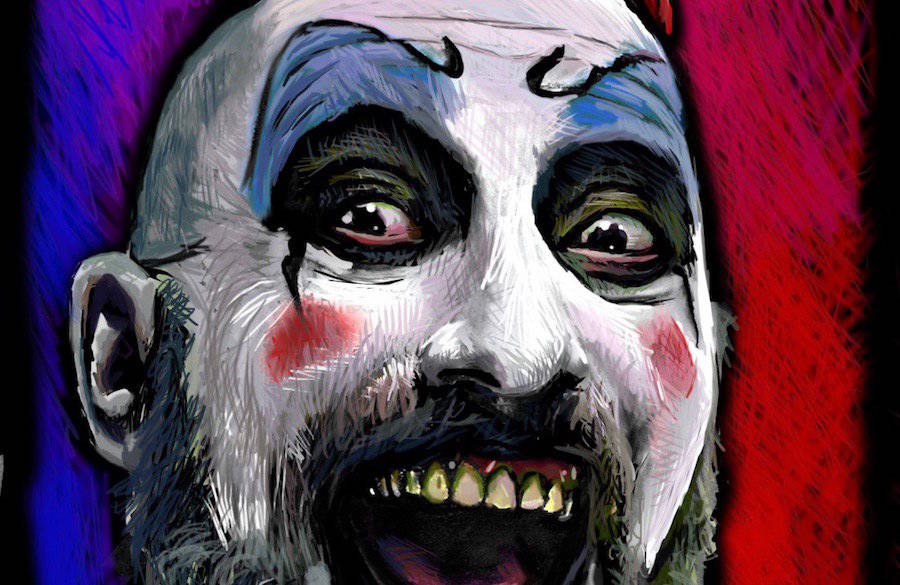This is a landscape-oriented painting featuring a sinister-looking clown face. The background consists of vertically arranged stripes in black, red, and blue colors. The clown's face is the focal point, centered within the composition, and it cuts off at the forehead, leaving only the top teeth visible due to the open mouth. The clown’s face is entirely painted white, with exaggerated black eyebrows and a startling mix of black and blue eyeshadow. The eyes, bloodshot with black pupils, are wide open, contributing to the menacing and evil expression. Additionally, there are red dots on the clown’s cheeks, and a distinct black mustache with a partially visible beard. The teeth are depicted as decayed, displaying an unappealing yellow-green hue, further enhancing the unsettling appearance. While the painting evokes discomfort, its details are meticulously crafted to create a chilling, impactful image.